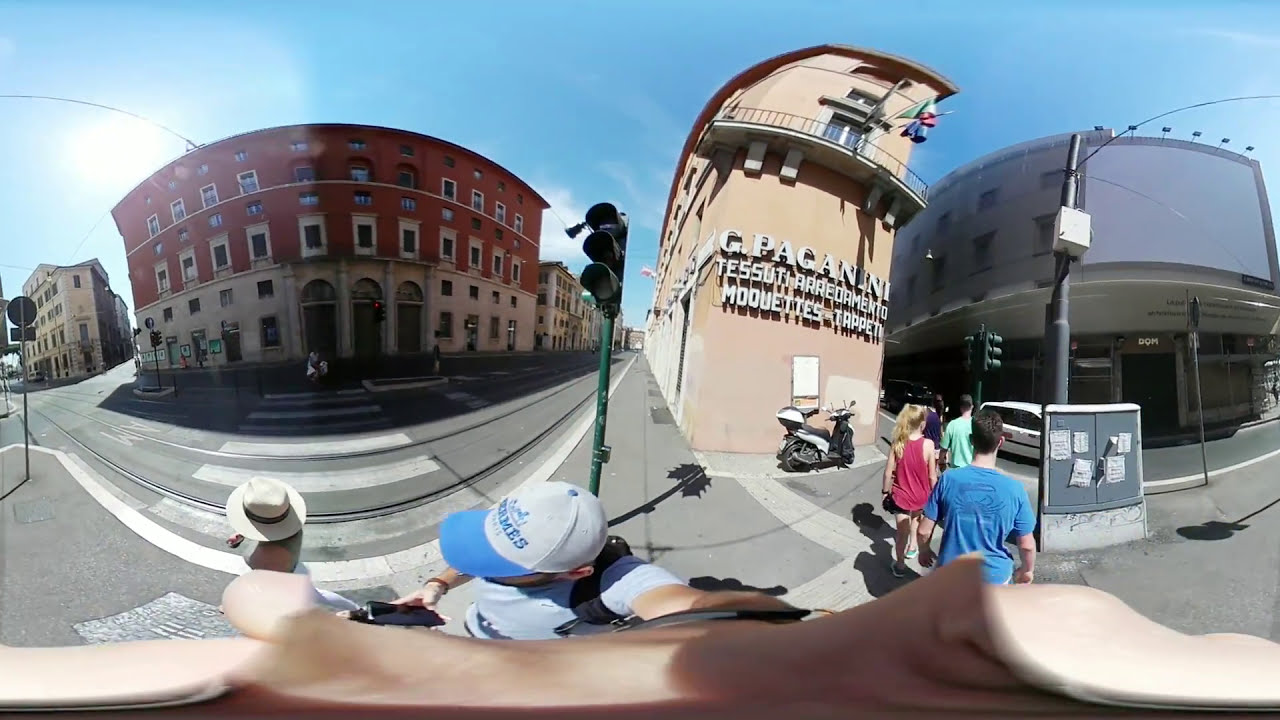The image captures a vibrant street scene in a charming commercial area that could be located in a small town either in the Northeastern United States or in Europe, possibly Italy. Dominating the center of the frame is a brick building with a stone base, exuding an old-world charm. Adjacent to it on the right is a building with the name "G Paganini," suggesting the setting might indeed be in Italy. Beyond this, there is a modern concrete structure, towards which a few pedestrians are crossing. 

Foregrounding the scene, taken with a fisheye lens, is a young man who appears to be taking a selfie. He wears a gray shirt, a white cap with a blue brim, and holds a smartphone. The wide-angle lens creates a dynamic, immersive perspective. Flanking him, people are going about their day: a young man in a blue T-shirt and a young woman in a red sweatshirt stand out as they cross the street, along with another young man in a light green shirt. Another young lady is visible to the left of the man taking the selfie.

The street itself is devoid of cars, amplifying the leisurely ambiance of this daytime scene. The sky above is mostly clear with a few light clouds, painted by the soft afternoon sun, suggesting it could be mid to late afternoon. The blend of historical architecture and daily life captures a moment that feels both timeless and contemporary.